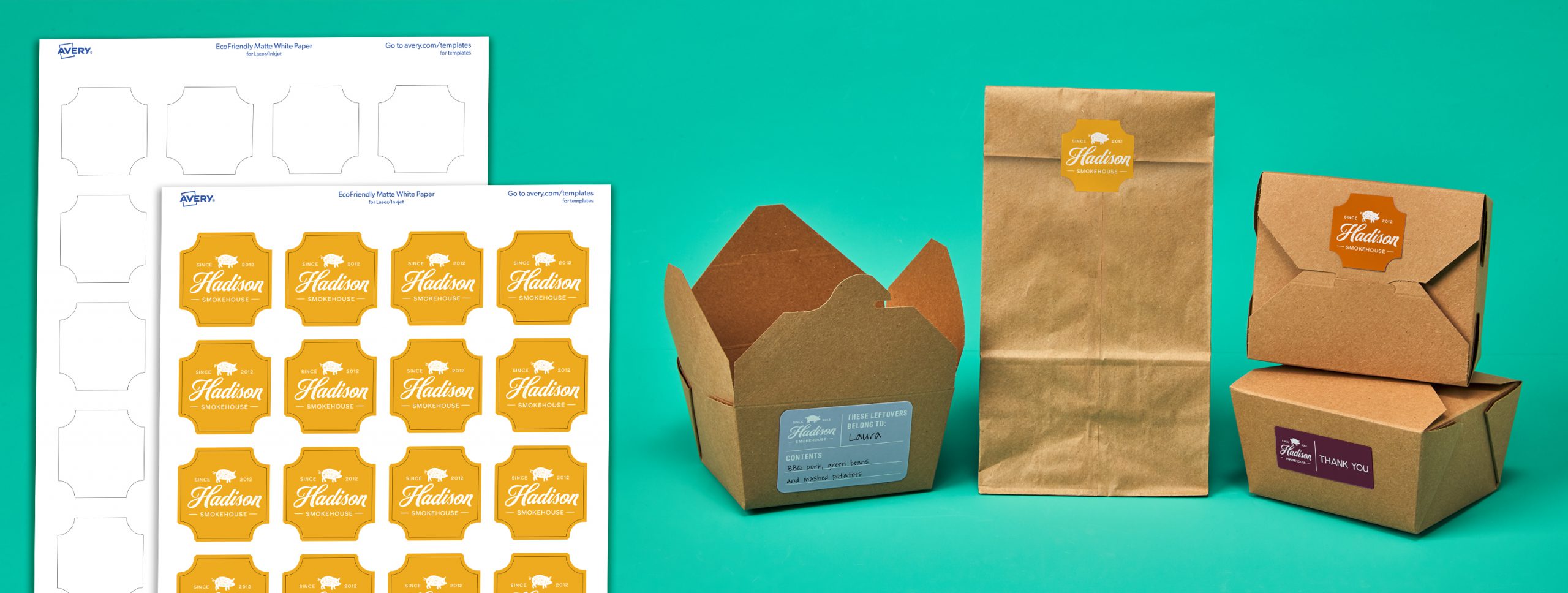The image features a horizontal rectangular graphic with a predominant teal or turquoise background. On the left side, there are two sheets of labels from Avery, a company known for paper and printing templates. The front sheet showcases gold stickers with concave corners that feature a central pig motif and text in various fonts. Surrounding the pig, "Since" is written on the left and "2012" on the right, with "Haddison" in large cursive white text beneath the pig and "Smokehouse" in smaller white text underneath that. The second sheet in the background matches the shape of the stickers but is blank.

On the right side of the graphic, practical applications for the labels are depicted. There are brown takeout containers and a brown paper bag, each adorned with Haddison Smokehouse labels. These labels are placed over the flaps of the containers and on the front of the paper bag, demonstrating their use in branding and identifying leftovers. Additionally, these labels prominently feature the same pig design and text detailing the establishment since 2012.